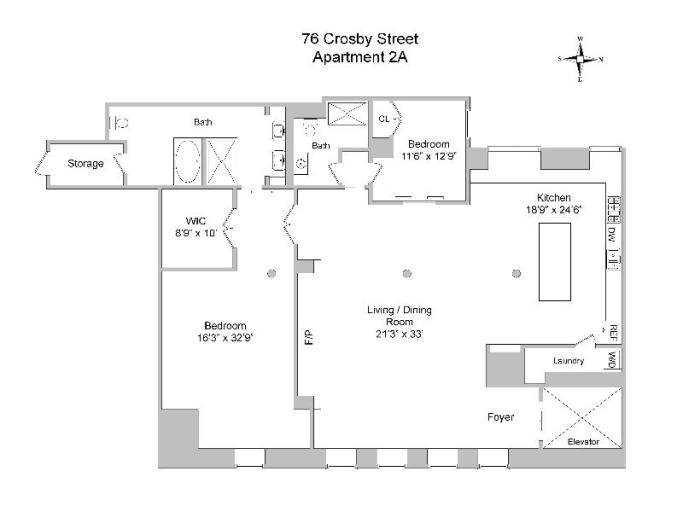This image depicts a detailed blueprint of an apartment located at 76 Crosby Street, Apartment 2A. The blueprint is rendered on a white background with light blue lines delineating the various rooms and spaces. 

In the top left corner, there's a small star-shaped compass indicating the cardinal directions: north, south, east, and west. To the left of the plan, there's a storage area leading into a bathroom equipped with a tub, a toilet, and a double sink. This bathroom is adjacent to a walk-in closet (WIC) measuring 8 feet 9 inches by 10 feet.

Next to it lies a generously-sized bedroom, spanning 16 feet 3 inches by 32 feet 9 inches. Opposite this bedroom is a combined living and dining room area, measuring 21 feet 3 inches by 33 feet, offering ample space for various activities and furnishings. 

The blueprint also features a foyer with an elevator for easy access to the apartment. Nearby, a compact laundry room houses a washer and dryer. The kitchen measures 18 feet 9 inches by 24 feet 6 inches and includes detailed placements of all appliances, including a dishwasher. 

Another bedroom, sized at 11 feet 6 inches by 12 feet 9 inches, also appears in the layout, accompanied by an adjoining half bath. 

This highly detailed floor plan provides a comprehensive overview of Apartment 2A at 76 Crosby Street, illustrating its spacious and well-organized living spaces.